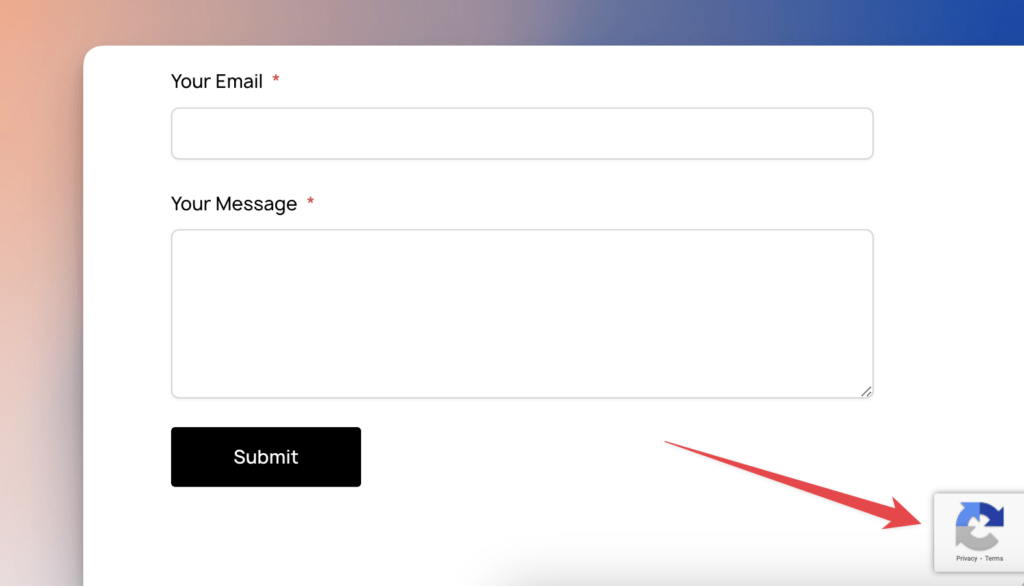The image is a colorful screenshot of a laptop screen, primarily showcasing a large, white pop-up window that occupies the majority of the screen, demanding the user's attention. The pop-up, essential for interaction, contains two fields denoted with mandatory red asterisks: one for the user's email address and the other for their message. The email address field is a single-line input, implying brevity, while the message field is a spacious multiline box, accommodating more extended responses. An arrow guides the user from their message to a CAPTCHA command situated at the bottom right, ensuring authentication.

Behind the prominent form, the background is a visually appealing, abstract gradient that transitions from warm orange hues on the left to cool blues on the right, adding a vibrant and modern touch to the image. Though the form dominates the view, this colorful backdrop subtly complements the functional design.